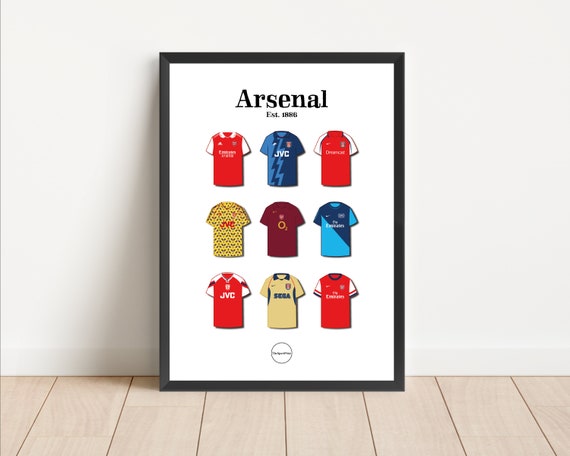This image depicts a sports-themed, framed art print showcasing a series of Arsenal football club jerseys. The print features a thin black frame and sits on a tan hardwood floor, leaning against a white wall with white molding at the bottom. The background of the print is white, and at the top, it prominently displays the word "Arsenal" in large black font, accompanied by "EST 1886" in smaller text below.

The illustration includes nine jerseys arranged in three rows. Each jersey exhibits different designs and sponsors over the years. The jerseys in the top row are, from left to right, a red one with white sleeves and collar, a blue one with "JVC" in white, and another red and white jersey. The middle row features a yellow jersey with a subtle pattern and "JVC 2," a maroon shirt with "O2," and a dark and light blue shirt possibly displaying "Emirates." The bottom row has a red jersey with white sleeves and "JVC," a yellow jersey with a blue collar that seems to read "SEAS," and a final red jersey with white sleeves and red and black striped cuffs, displaying "Emirates." The entire illustration is masterfully framed in a thin black frame, adding a touch of elegance to its display.